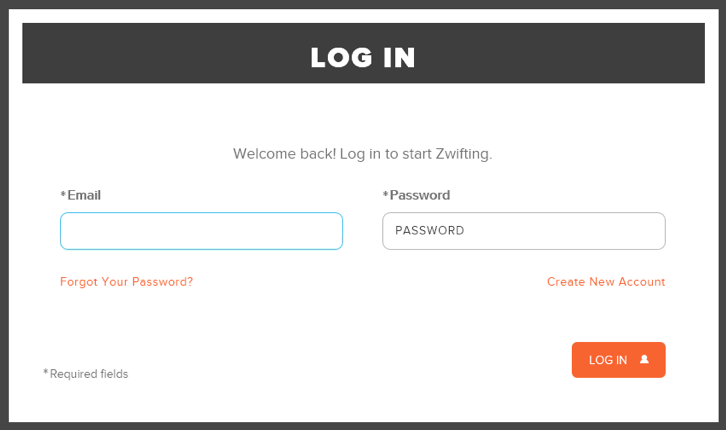The image depicts a login interface for Zwift, presented on a clean white background with a black outline. At the top, the text "Login" is prominently displayed in white. Below that, the phrase "Welcome back! Log in to start Zwifting" invites users to access their accounts.

Users are prompted to enter their credentials, starting with an email address in a designated box labeled "Email." Below this, there's a "Forgot your password?" link for those who may need to recover their login information. Next, there's a section for "Password," followed by another input box labeled "Password."

Underneath the password box, a "Create new account" option is provided for new users. To the bottom right, an orange box featuring a person symbol and the text "Log in" serves as the final step for logging in.

A small symbol of a star in the corner, accompanied by the text "Required fields," indicates that the email and password fields are mandatory for logging in.